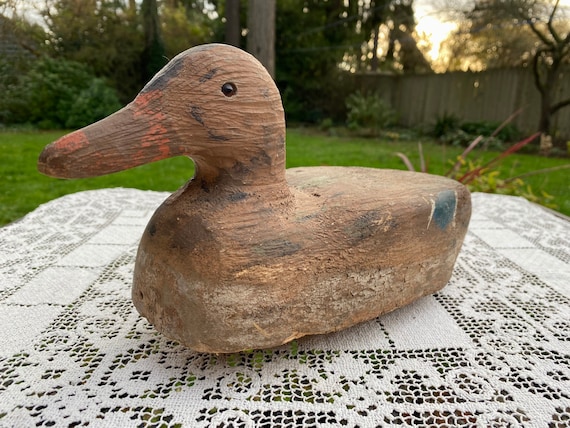This photograph captures a rustic, handcrafted wooden duck prominently displayed at the center of a square table draped with an intricate white lace tablecloth or doily. The wooden duck, weathered and muddied, has a rich brown body and glass eyes, with an orange beak that is largely obscured by dirt and wear. Positioned in an outdoor setting, the scene is framed by a well-kept green lawn, a wooden fence, and a variety of trees and shrubs. In the background, between the greenery, you can catch a glimpse of a soft orange sunset sky, adding a serene ambiance to the image. The duck, with its traditional design and age-old charm, commands the viewer's attention while the detailed lacework beneath it complements the rustic feel of the picture, which appears to be taken in someone's personal backyard.